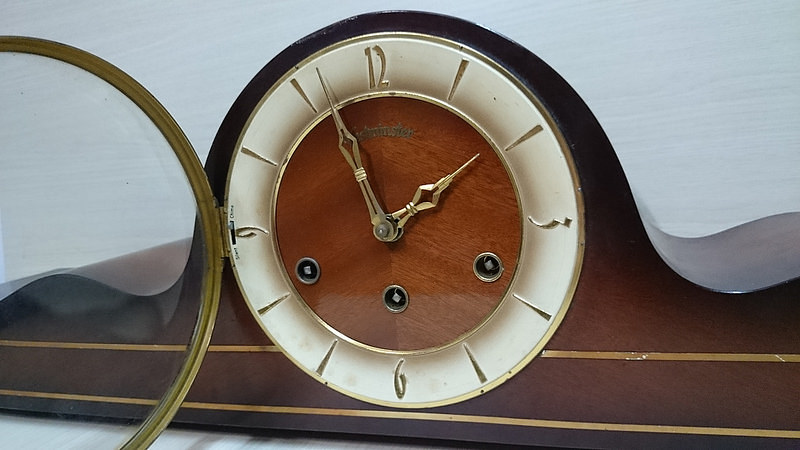This is a detailed photograph of an antique wooden clock with an elegant, polished finish. The clock features a distinctive design with a flat base and sides that gracefully curve upwards like waves toward the circular center, which houses the clock face. The clock has a glass door with a gold rim that is fully open to the left in the image, revealing the face of the clock clearly.

The face of the clock is adorned with golden numbers and hands, which are intricately designed. The numbers 3, 6, 9, and 12 are prominently displayed in a golden hue around a white ring, making them easy to read. The remaining hours are indicated by gold hash marks. The center of the face is dark brown, providing a striking contrast to the white ring and gold details. The time on the clock appears to be set to 1:57.

Additionally, the clock has three round screw areas and two gold lines that run along the lower part of the clock, adding to its decorative elements. The background features a grayish-white painted wall, subtly emphasizing the rich details of the wooden clock in the foreground.